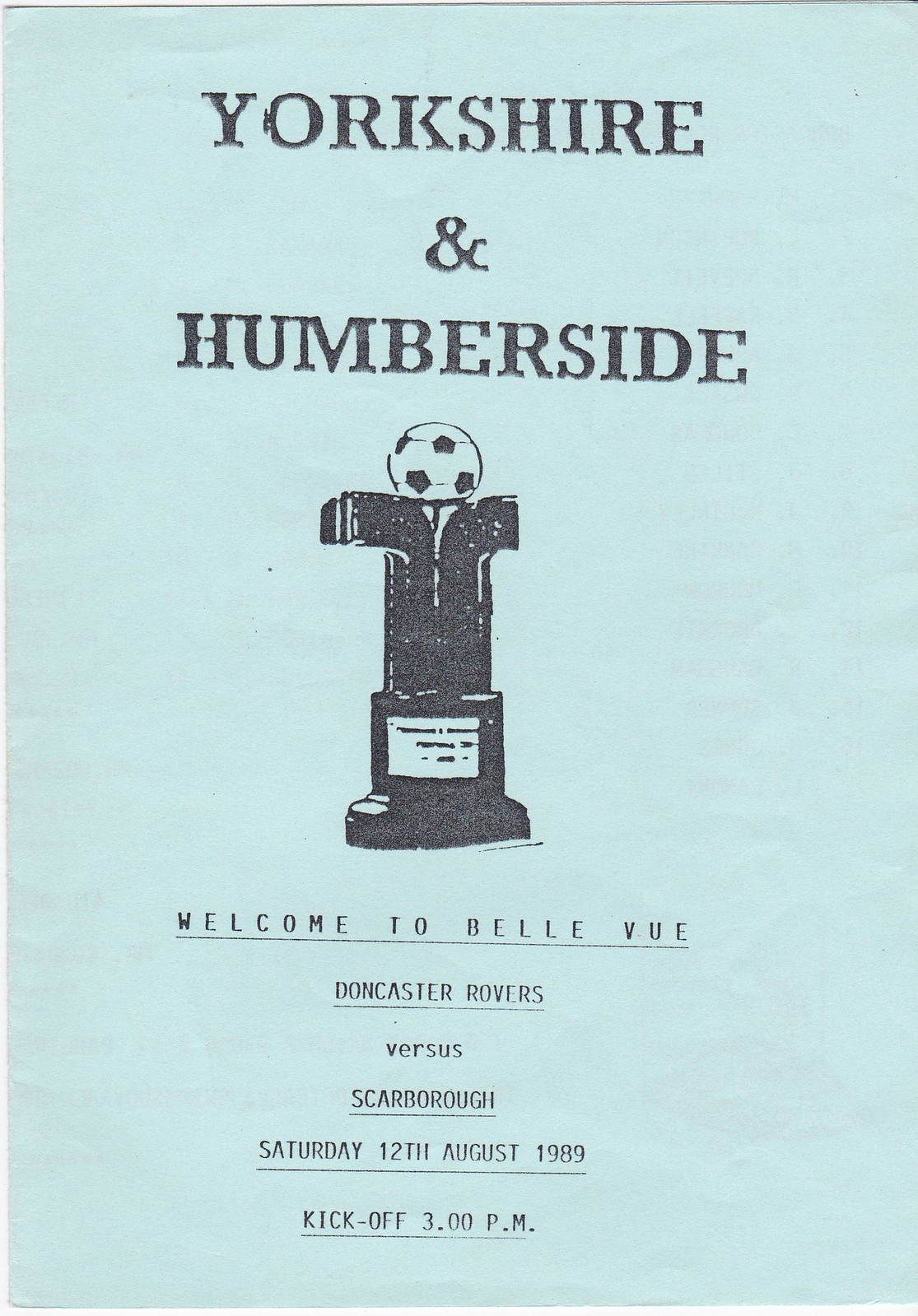This image depicts an aged, light blue flyer or program cover with a black print, likely from a sporting event. At the top, in large, capitalized font, are the words "YORKSHIRE & HUMBERSIDE." Directly beneath this, there is an illustration of a trophy supported by shapes resembling inverted J's, with a soccer ball perched on top and a circular base below. Following the graphic, the text continues with, "Welcome to Bellevue," "Doncaster Rovers versus Scarborough," all underlined, and concludes with "Saturday 12th August 1989" and "kickoff at 3 o'clock p.m.," also underlined. The overall appearance suggests it is an old, photocopied document, centered and neatly arranged.